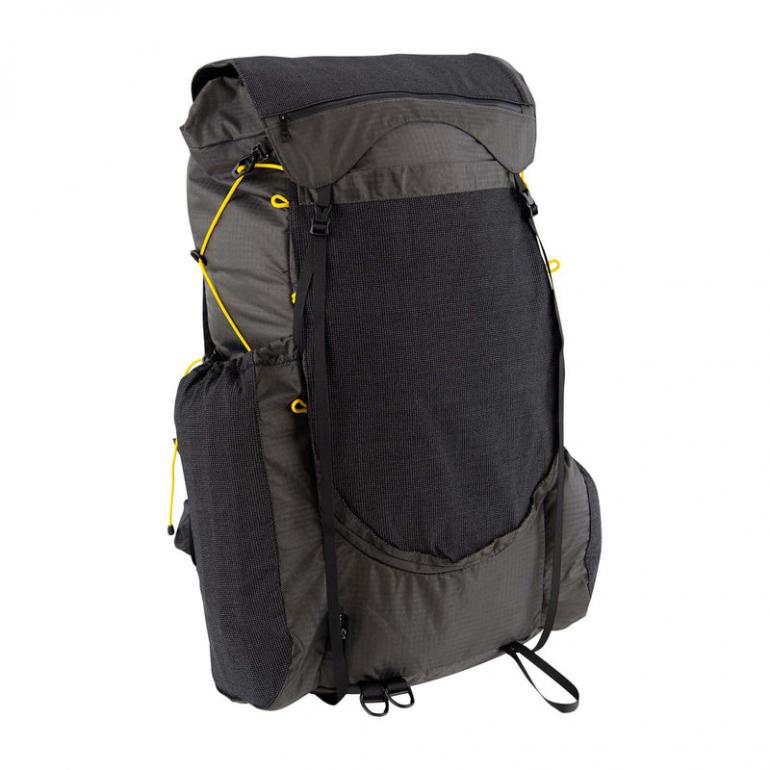This image features a dark-colored backpack prominently displayed against a white background, highlighting its intricate details without any distracting elements. The backpack is predominantly composed of sections that alternate between a dark charcoal gray and nearly black hues, with subtle hints of a pale light greenish gray. Notably, it has gold or light yellow strings and bands on the sides and bottom, likely for attaching or securing additional items, enhancing its utility for camping or long trips.

The backpack is of a substantial size, structured in a rectangular, or portrait orientation – taller than it is wide. At the top, a horizontal zipper allows for easy access to the main compartment. The design includes a fold-over top that clips down into a black circular or oval shape, providing extra security for the contents. There are two black clips on the left and one on the right, partially hidden by bulging side pockets that hint at ample storage space and potentially elastic material for expansion.

The bottom section features small rings and a plastic loop, which suggest multiple purposes, from attaching gear to allowing it to be strapped down securely. The backpack also includes black straps, likely adjustable, further indicating its suitability for carrying heavier loads over long distances. This detailed and well-constructed design emphasizes the versatility and practicality of the backpack, perfect for outdoor adventures.